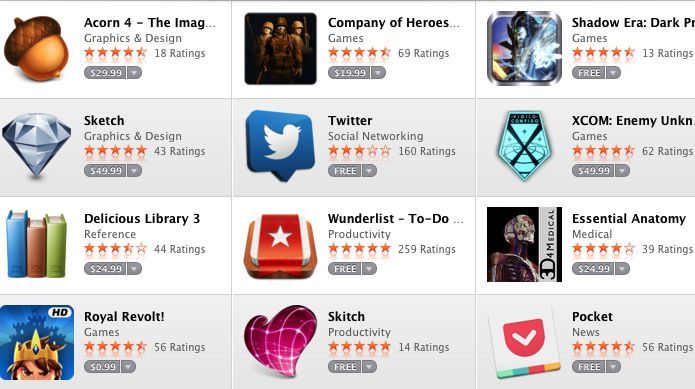The image depicts a rectangular grid divided into 12 squares, organized in four rows of three columns each. Each square showcases an icon and details of different apps or games:

1. **Top Left Square:** 
   - **Icon:** Acorn.
   - **Name:** Acorn4.
   - **Description:** acorn4 dash, then I-M-A-G ...
   - **Price:** $29.99.

2. **Top Middle Square:**
   - **Name:** Company of Heroes.
   - **Rating:** 5 stars.
   - **Price:** $29.99.

3. **Top Right Square:**
   - **Name:** Shadow Era: Dark ...
   - **Description:** shadow era colon dark P-R ...
   - **Rating:** 4.5 stars from 13 ratings.
   - **Price:** Free.

4. **Second Row, Left Square:**
   - **Name:** Sketch.

5. **Second Row, Middle Square:**
   - **Name:** Twitter.

6. **Second Row, Right Square:**
   - **Name:** XCOM: Enemy …
   - **Description:** xcom colon enemy U-M-K-A-N.

7. **Third Row, Left Square:**
   - **Name:** Delicious Library 3.

8. **Third Row, Middle Square:**
   - **Name:** Wonderlust-2-Do.

9. **Third Row, Right Square:**
   - **Name:** Essential Anatomy Medical.

10. **Bottom Row, Left Square:**
    - **Name:** Royal Revolt!
    - **Icon:** Marked HD.

11. **Bottom Row, Middle Square:**
    - **Name:** Sketch Productivity.

12. **Bottom Row, Right Square:**
    - **Name:** Pocket News.